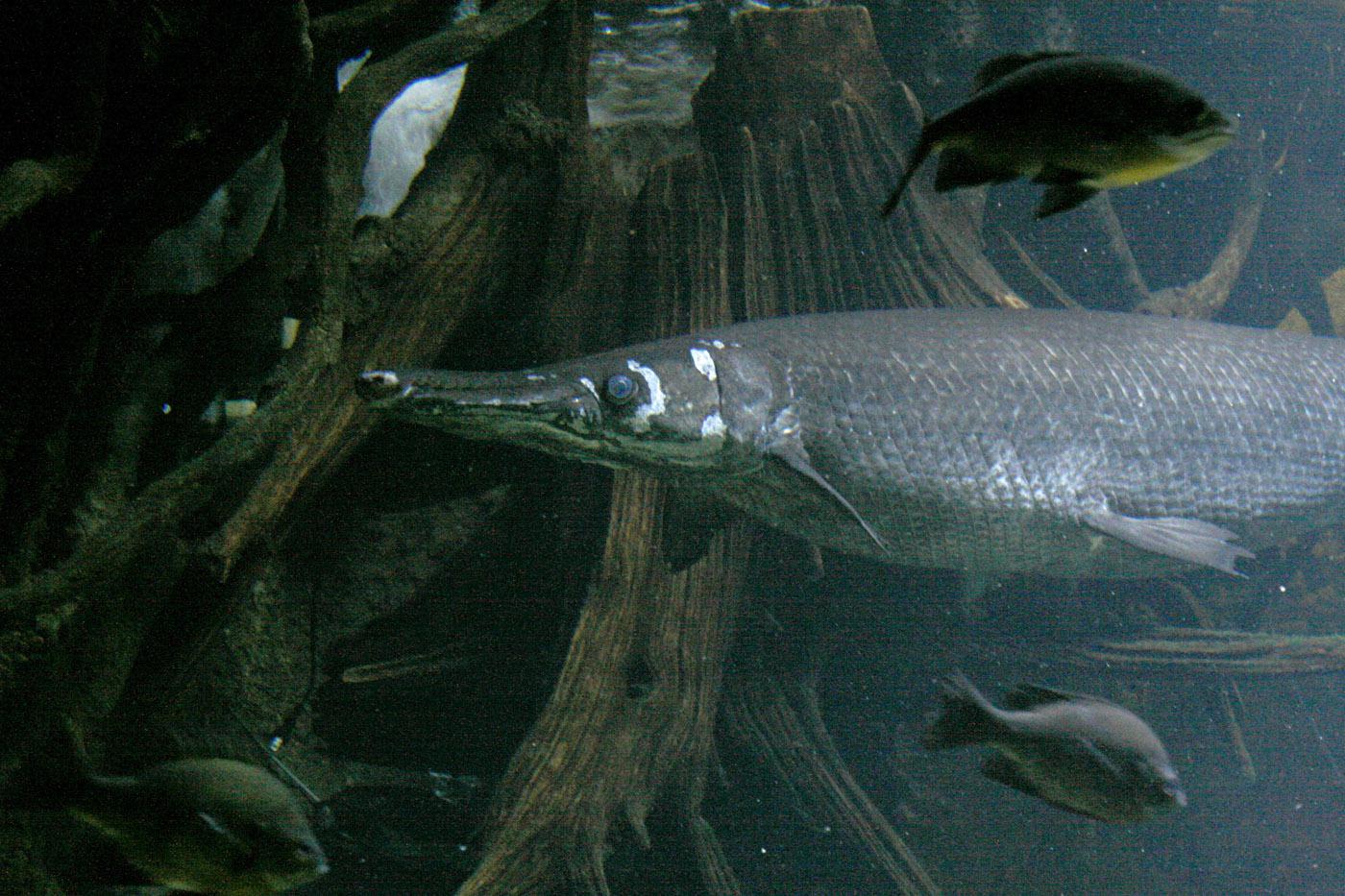This photograph portrays an underwater scene dominated by four distinct fish, swimming around what appears to be the submerged roots of a disintegrating tree stump. The focal point of the image is an unusual gray fish with a remarkably long, slim mouth and a sizeable eye, identified as possibly a gar. It occupies the center of the picture, positioned near the tree stump's base. Above this gar-like fish, a smaller fish with a yellowish belly and greenish tint swims in the opposite direction, facing to the right. Below, closer to the bottom of the image, a small gray fish heads towards the bottom right corner. Additionally, there's another small fish in the bottom left, also facing right. The scene is captured in murky waters dominated by dark greens and grays, with a noticeable gap at the top of the photo revealing a glimpse of the water's surface. The overall ambiance is shadowy and subdued, emphasizing the mysterious environment these fish inhabit.